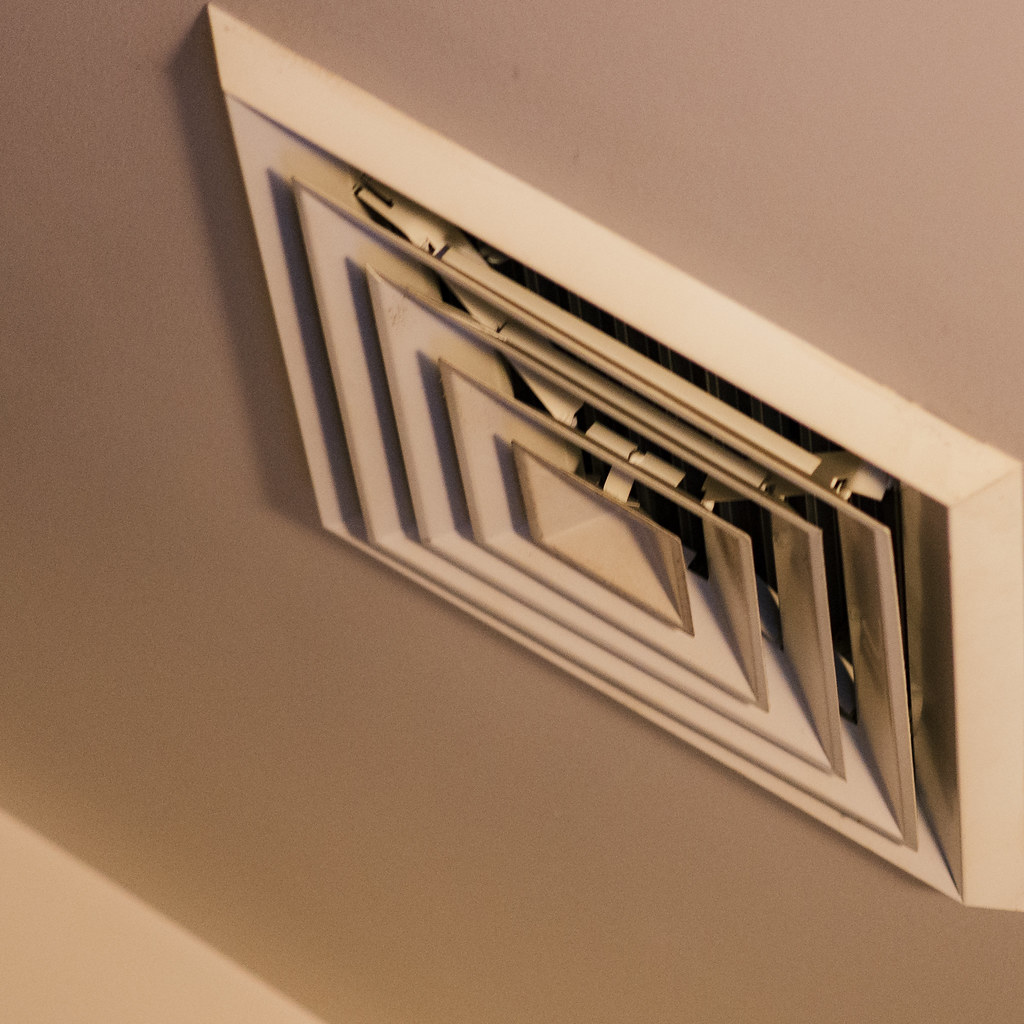The image depicts a zoomed-in view of a square ceiling air vent, centrally positioned against a light to dark brown background. The ceiling, captured at a diagonal angle with its highest point on the left, slopes gently downward to the right. The vent, possibly made of plastic, features a series of progressively smaller squares within its frame, creating a layered, grid-like appearance, hinting at an intricate air filtration system. There are no people present in the image, allowing the focus to remain on the vent and its functional yet minimalist design. The lighting is minimal, highlighting the vent's ivory color against the contrasting brown tones of the ceiling, adding depth and dimension to the scene.